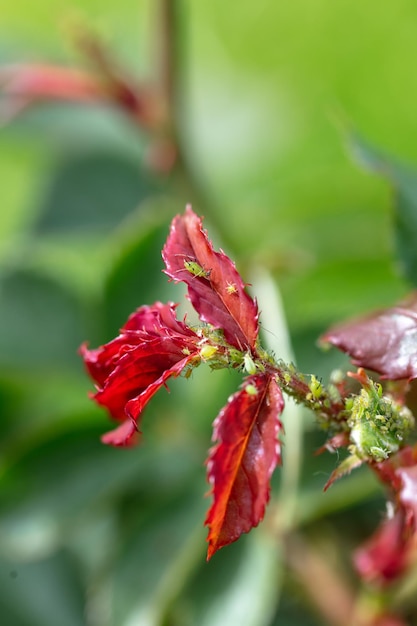This close-up photograph features a striking red flower as the central focus, distinguished by its spiky appearance and somewhat fuzzy, thorny red stem resembling a pipe cleaner. Three prominent red petals are clearly visible in the center, with additional petals becoming blurry towards the right. Several small, lime green or neon green bugs, marked with black specks, are scattered across the flower and stem, nestled in the crevices. The background is a soft blur, showcasing another red flower and an assortment of green leaves, imbuing the image with a lush, natural ambiance. The overall clarity and detail of the foreground contrast beautifully with the indistinct greenery behind.